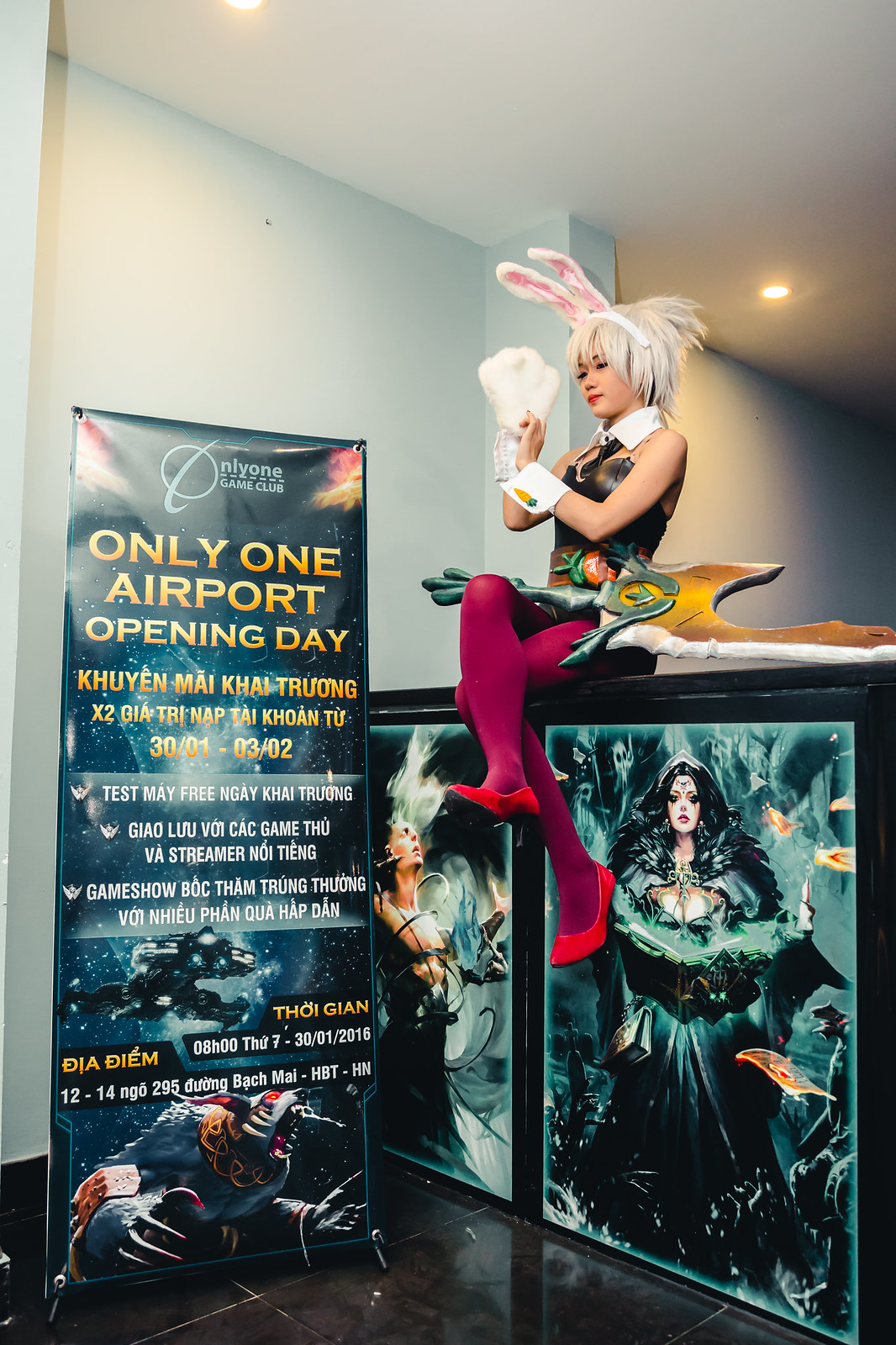In this full-color indoor photograph, a young woman dressed up for a cosplay event sits confidently on a ledge or booth. She sports a distinctive outfit: platinum blonde hair beneath oversized bunny ears, a black leather top with white cuffs, a white collar, a tie, and striking purple nylons paired with vibrant red shoes. A large toy sword rests across her lap. Behind her, the wall displays two posters, one featuring a man and the other a woman adorned in fantasy attire, suggesting an action-adventure theme. To her left is a prominent stand-up banner against a blue, starry backdrop, proclaiming "Only One Airport Opening Day," with additional script likely in Vietnamese. The floor beneath her is sleek black marble, adding an elegant touch to the ambiance that may well be part of a comic convention setting in Asia.